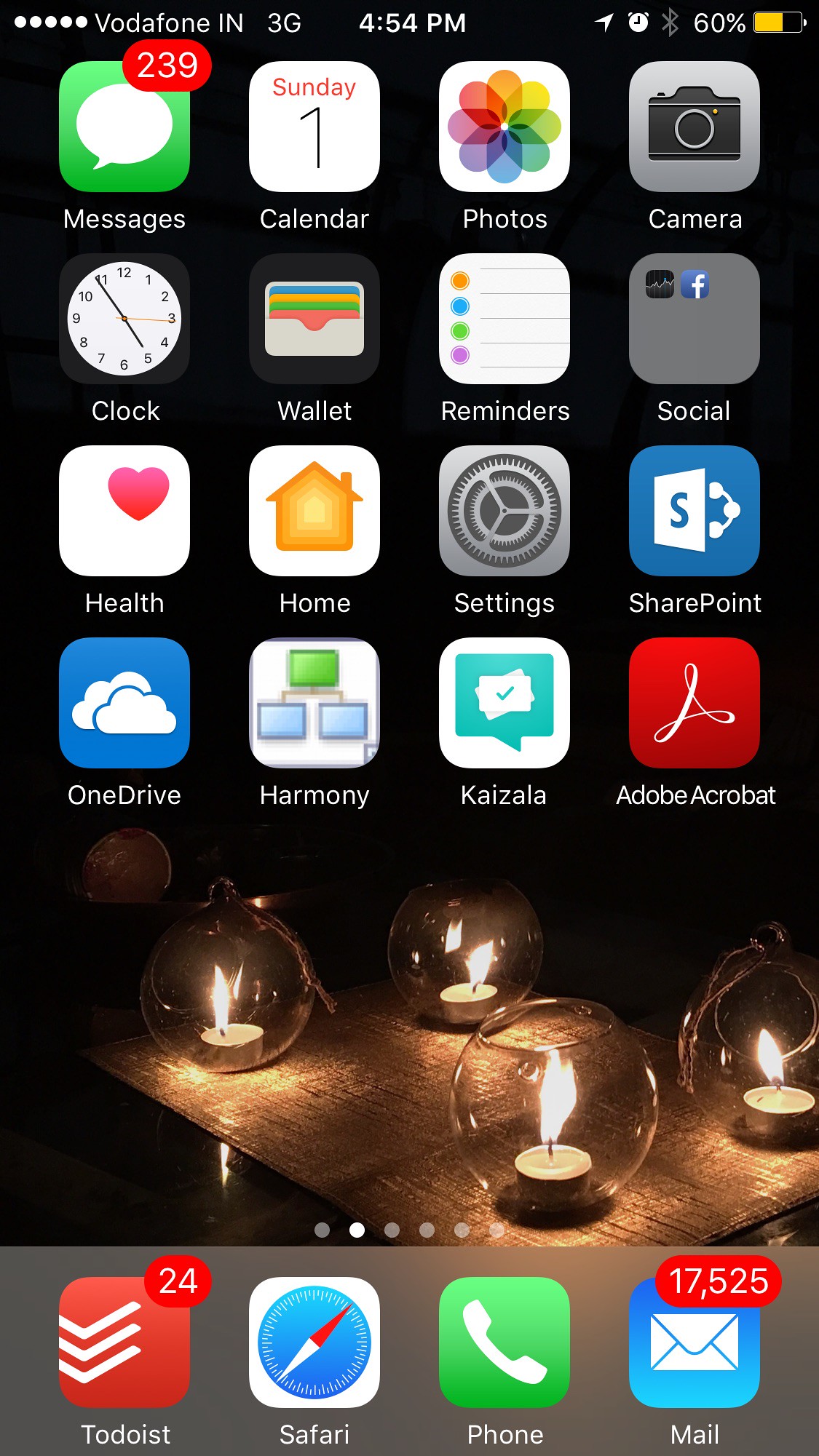The screenshot displays the home screen of a Vodafone smartphone connected to Vodafone IN 3G network. The status bar at the top shows the time as 4:54 p.m. and the battery level at 60%. 

The background image is of a table adorned with tea lights in glass globes, adding a warm and cozy ambiance to the screen. 

The bottom dock features icons for Todoist (with 24 pending alerts), Safari, Phone, and Mail (showing a staggering 17,525 unread emails). 

The home screen is populated with various apps, each serving different functions. The Messages app has 239 unread messages, and other visible apps include Calendar, Photos, Camera, Clock, Wallet, Reminders, Social, Health, Home, Settings, SharePoint, OneDrive, Harmony, Kaizala, and Adobe Acrobat. Additionally, there is an alarm set, as indicated by an icon in the status bar at the top. 

This detailed depiction highlights the smartphone's activity and the user's engagement with multiple applications and pending notifications.